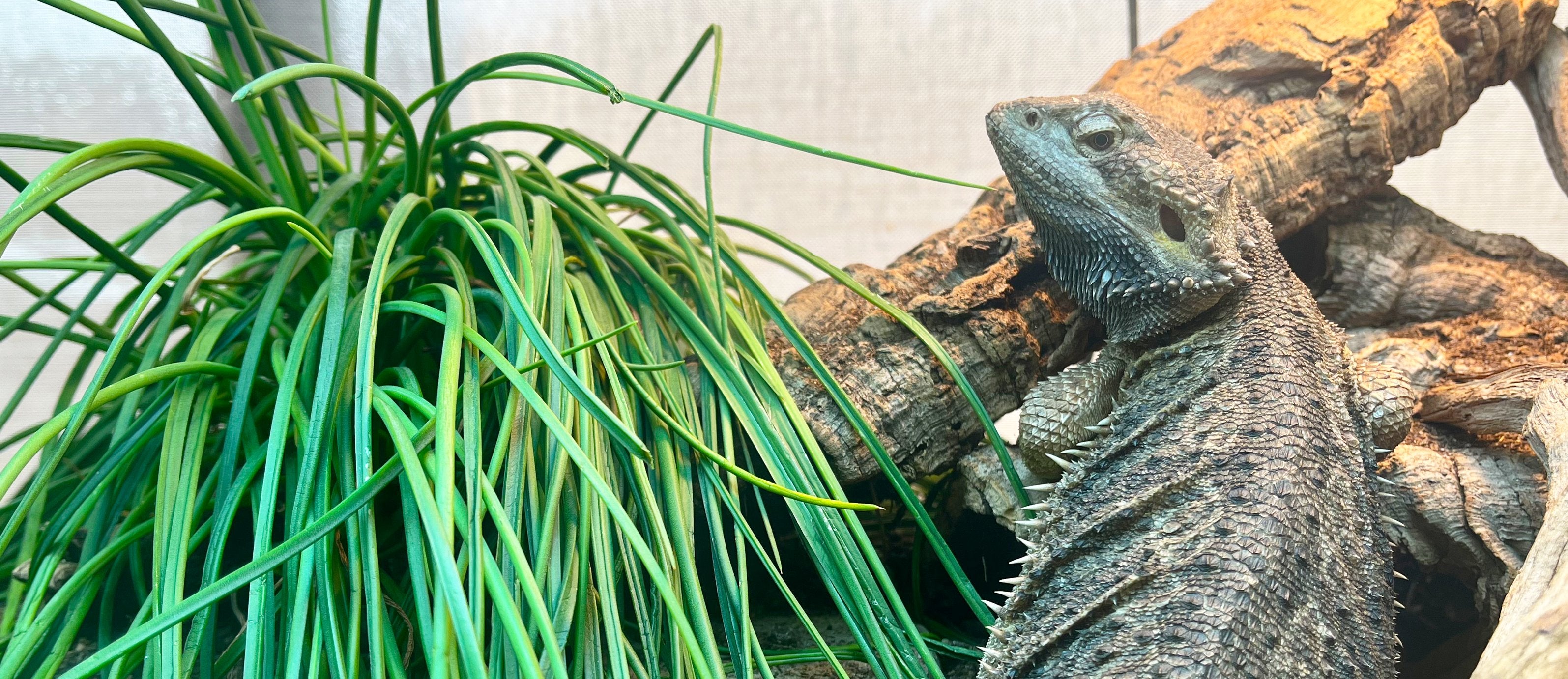This photograph captures a bearded dragon, predominantly gray with hints of white and brown and adorned with sharp white spikes along its sides. The reptile is positioned on the right side of the image, resting on an angled wooden branch that descends from the top right toward the left. Its body faces away from the camera, while its head is turned back, giving a clear view of the left side of its face. Warm light illuminates the dragon and the wood beneath it. To the left, a vibrant, green pom-pom-shaped foliage with thick, stringy leaves contrasts against the reptile. The beige background features a blurred white mesh or blinds, suggesting the setting is a terrarium within a house, likely captured during the day.